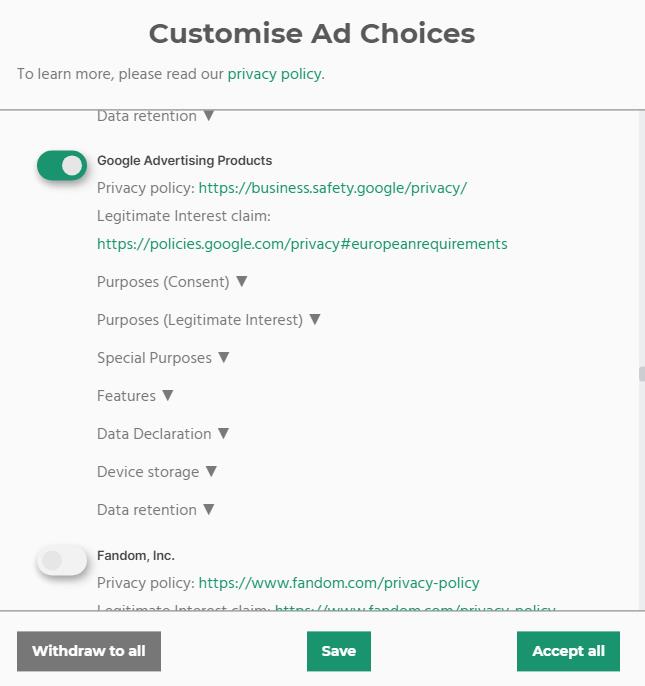This detailed screenshot features an off-white background. At the top, prominently displayed in large, bold, dark gray letters, is the heading: "Customize, Add Choices." Directly beneath this, in a smaller font, is the message: "To learn more, please read our privacy policy," with the phrase "privacy policy" highlighted in green.

A thin gray line separates this section from the subsequent content. Below this line, additional text lists key topics: "Data Retention, Google Advertising Products, Privacy Policy, Legitimate Interest Claim." After the phrases "Privacy Policy" and "Legitimate Interest Claim," there are accompanying URLs presented in green text. 

Alongside the term "Google," there is a small green toggle button that is currently toggled on. Further down, the text lists several categories with small arrow triangles next to each one: "Purposes, Consent, Purposes, Legitimate Interest, Special Purposes, Features, Data Declaration, Device Storage, Data Retention."

Below these categories, the text "Fandom Incorporated" is displayed with a small button next to it that is toggled off. 

At the very bottom of the screen, three rectangular buttons are visible. The buttons labeled "Save" and "Accept All" are green, while the button labeled "Withdraw to All" is not highlighted in green.